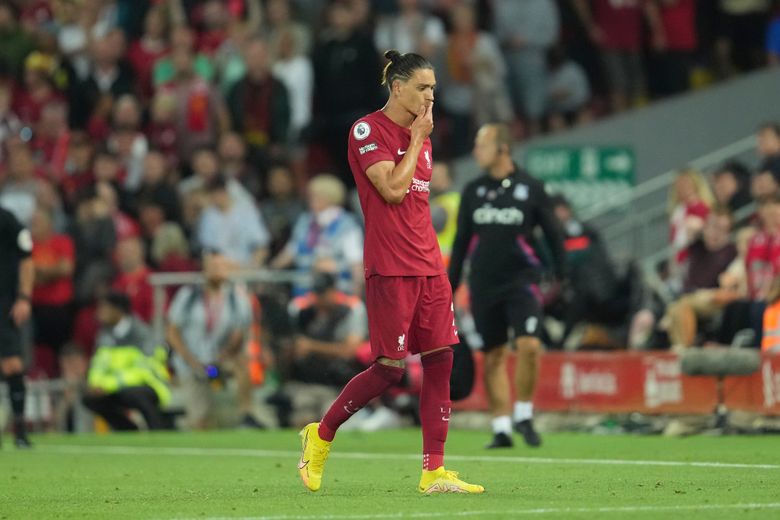The photograph captures a soccer player, deep in thought, with his hand covering his mouth, walking across a grass field that appears to be astroturf, given its light green color with white lines. He is outfitted in a complete maroon uniform, including a maroon jersey with a visible Nike swoosh, maroon shorts, and maroon socks pulled above the knee. His striking yellow athletic shoes stand out vividly. His hair is pulled back into a bun on top of his head. In the background, an opposing team player is dressed entirely in black, from his jersey to his shorter socks and black shoes. Beyond them, out of focus, spectators fill the stands, their attention directed elsewhere, presumably towards recent on-field action. Some spectators are also visible below the stands, donning reflective gear, emphasizing the bustling atmosphere of the setting. The scene suggests a moment of reflective pause for the maroon-clad player amidst the dynamic backdrop of the match and its audience.